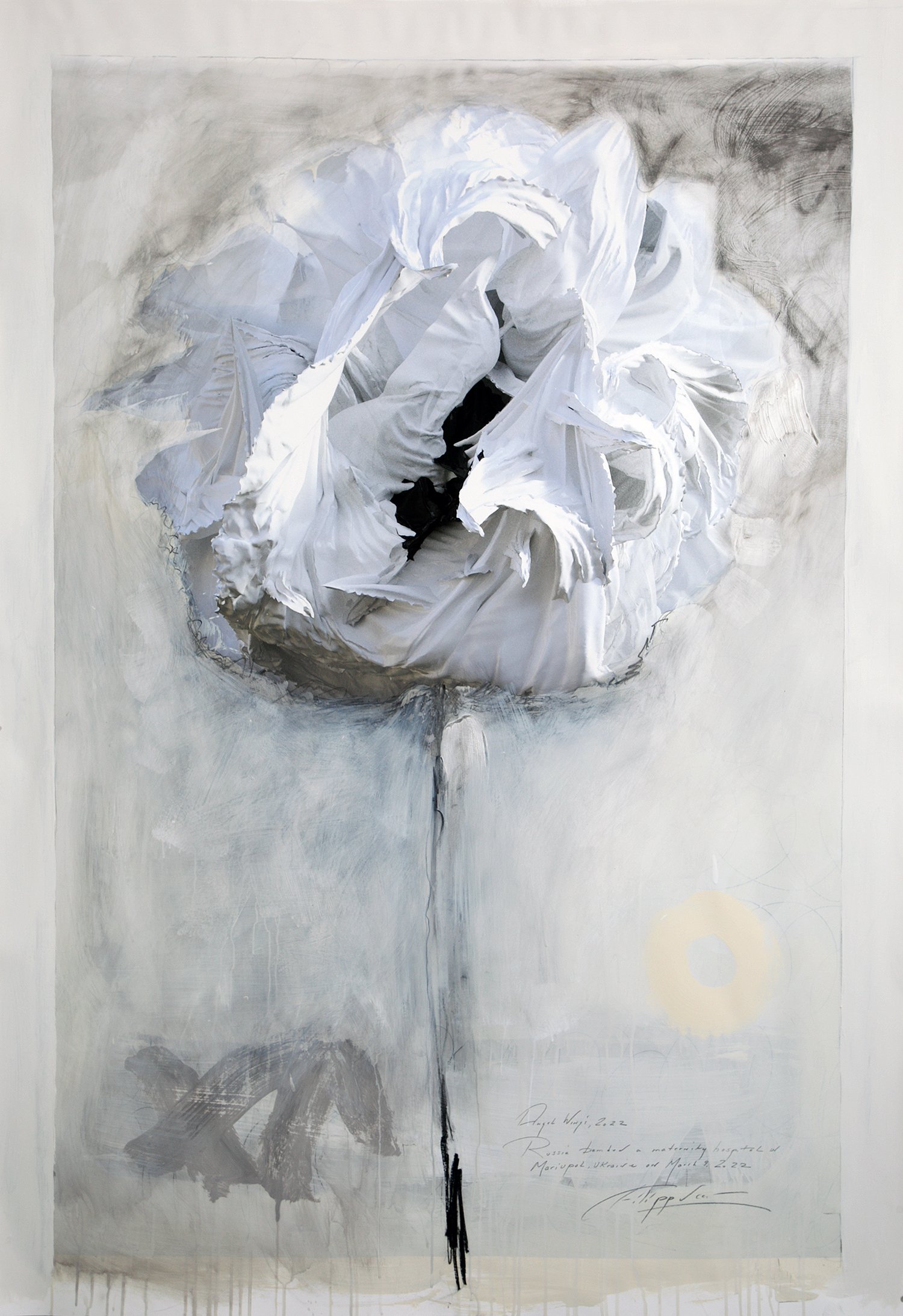In this abstract artwork, we observe a predominantly black and white composition with accents of beige, milky, and peach colors. At the center of the image, there is a feature that vaguely resembles a white flower or a piece of white clothing, with a swirling texture built up around it. This central area seems to create a black hole-like space in the middle. A black stalk-like structure extends from the bottom to the top of the image, intersecting the swirling white area. Towards the bottom right of the picture, there is faint writing and a signature, though it is difficult to decipher. Additionally, the background includes various shades of white and gray, with darker black and gray strokes visible towards the top. On the left side of the image near the bottom, there seems to be an abstract structure, perhaps suggesting a caricature of a person walking on a road, accompanied by a symbol that looks like the letter "X". This eclectic composition leaves much to the viewer's interpretation, blending floral-like elements with abstract forms and subtle textual hints.